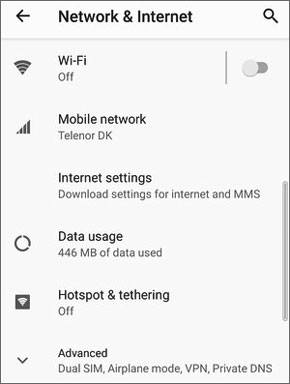The image captures a black-and-white interface of a phone's network and internet settings. At the top of the screen, the header reads "Network & Internet," followed by a search bar. Below, there's a section for Wi-Fi, displaying a Wi-Fi symbol and the status "Wi-Fi off," with a toggle switch set to the left indicating it is turned off.

Beneath the Wi-Fi section, the next entry shows "Mobile Network" with a four-bar signal icon and the text "Telenor DK." Further down, the "Internet Settings" option is available, allowing for the download of settings for internet and MMS.

Subsequently, the data usage for the phone is detailed, indicating "446 MB of data used" accompanied by a refresh symbol to update this information. Below this, a small Wi-Fi icon in black highlights the "Hotspot & Tethering" feature, currently marked as off.

At the bottom of the screen, there is an "Advanced" section, listing options such as "Dual SIM," "Airplane Mode," "VPN," and "Private DNS." Finally, along the right side of the page, there is a vertical scrollbar indicating the user's position within the settings menu.